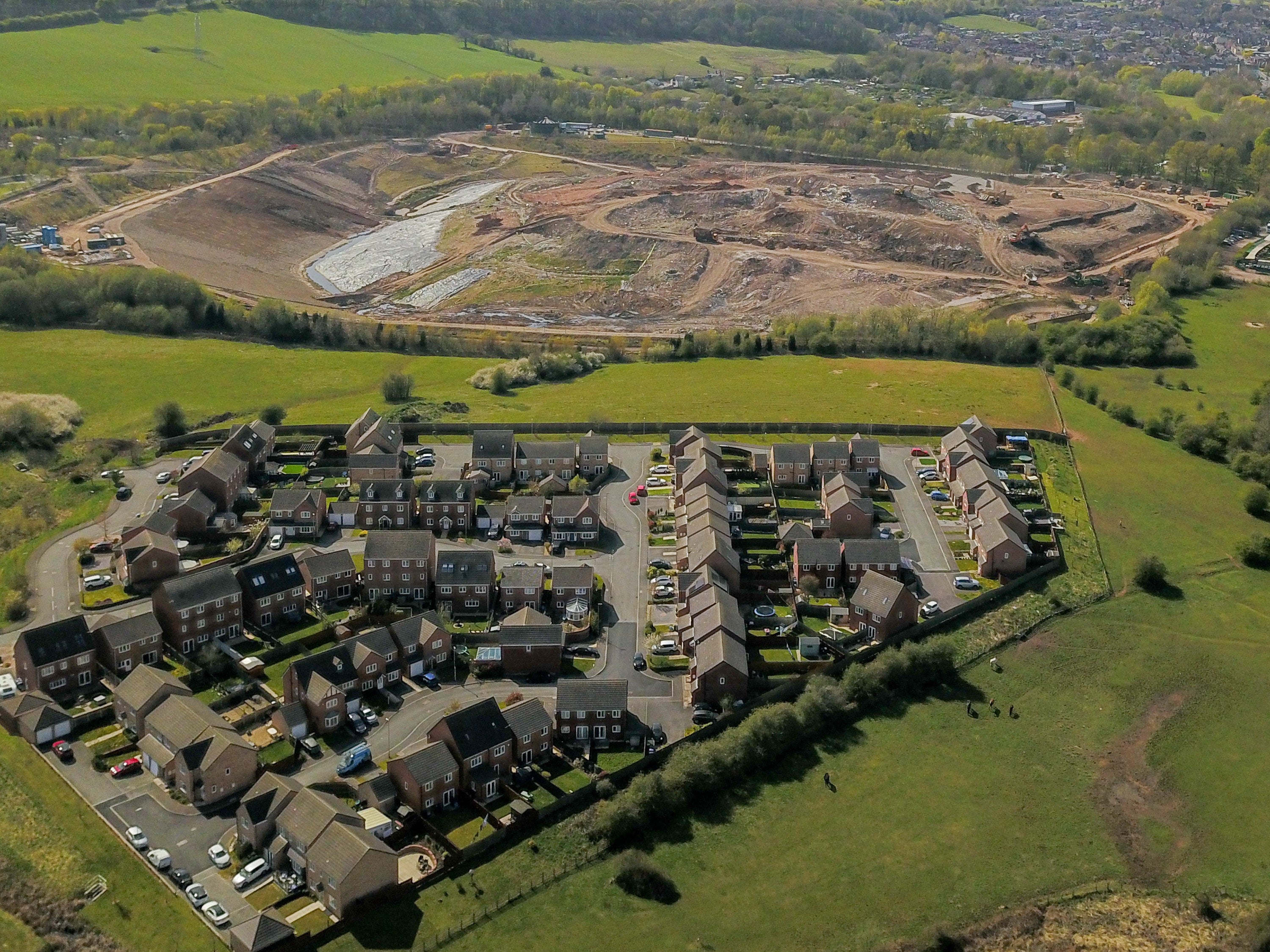This aerial drone photograph offers a comprehensive view of Elan Mas, showcasing a small city or town with neatly arranged houses that appear uniform in their dark brown hues and square shapes, many with dark brown roofs. The layout of the development resembles a triangular or arrow shape, with the wider end on the left narrowing to a point on the right, featuring paved roads throughout. Several cars of various colors, including white, blue, and red, are parked at various points in the town. The image captures people on the well-kept lawns, further bringing the scene to life.

Surrounding the town are expansive green fields dotted with shrubs and short grasses, creating a picturesque border. Towards the top of the photograph, in the background, there is a visible mining or construction site, with multiple roads weaving through dips in the terrain, suggesting active development. Heavy equipment such as backhoes is visible, along with sections of exposed dirt, indicating ongoing work. Beyond this area, a dense row of trees and bright green fields stretch into the horizon. Further in the distance, towards the top-right corner, another town is faintly visible, adding depth to the sprawling landscape.